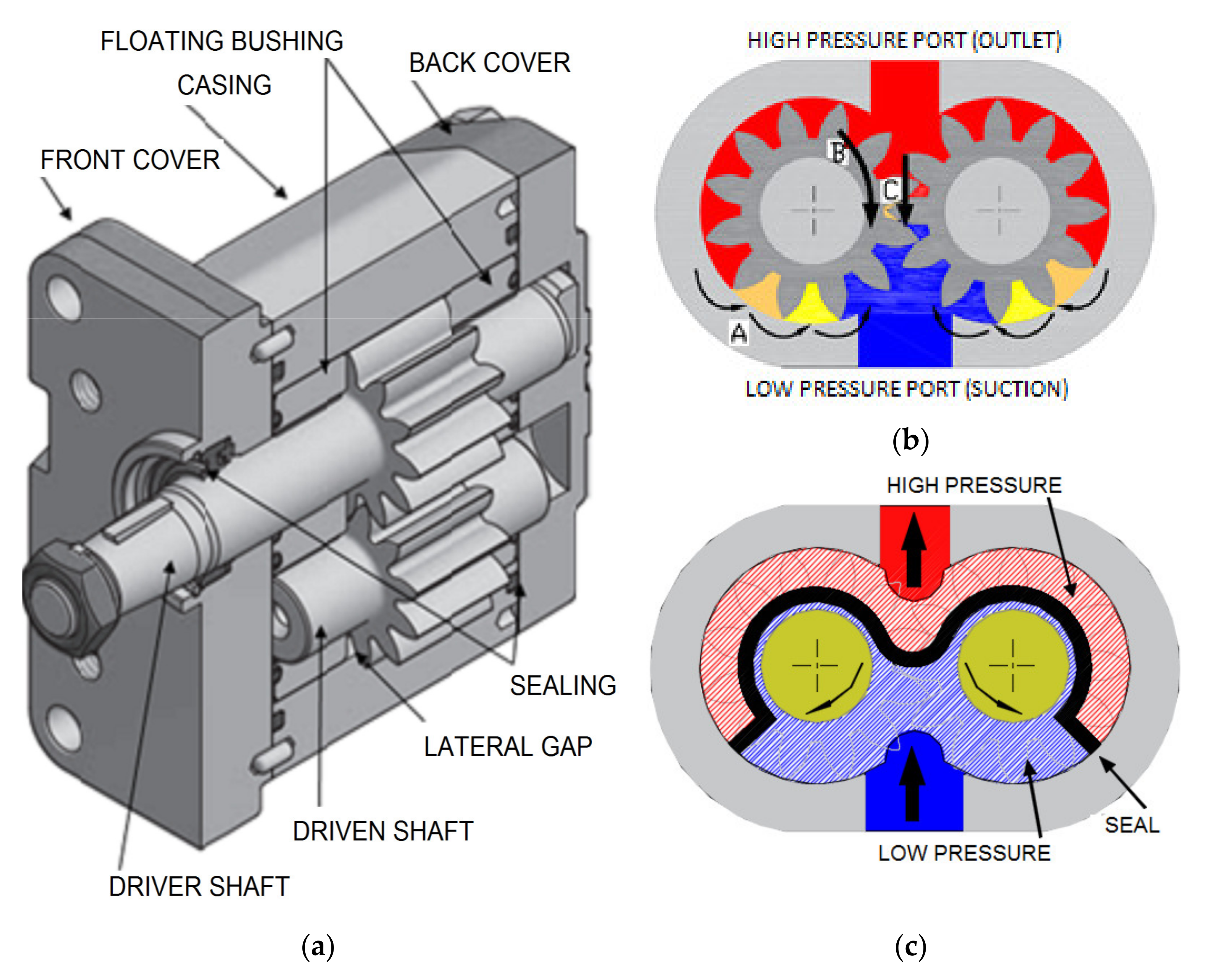The image is a detailed diagram that appears to be part of an instructional manual for a machinery component. The diagram is divided into three labeled sections: A, B, and C. 

On the left side of the diagram, section A depicts the exterior of a mechanical apparatus with key parts labeled, including a front cover, floating bushing casing, back cover, driver shaft, driven shaft, lateral gap, and sealing. The apparatus seems to be composed of metal and demonstrates various mechanical elements essential to its function.

To the right, section B provides an interior view of the apparatus, highlighting key pressure points. The labeling indicates a high-pressure port outlet at the top and a low-pressure port suction at the bottom. It also illustrates two circular components in proximity, visually linked with directional annotations.

Finally, section C, beneath section B, offers another internal perspective, accentuating the pressure dynamics. It is labeled with 'high pressure' at the top, 'seal' in the middle, and 'low pressure' at the bottom, correlating to the color-coded pressure zones throughout the apparatus. The diagram uses colors such as red, blue, yellow, and grey to delineate different pressure regions and components, enhancing clarity and detail for instructional purposes.